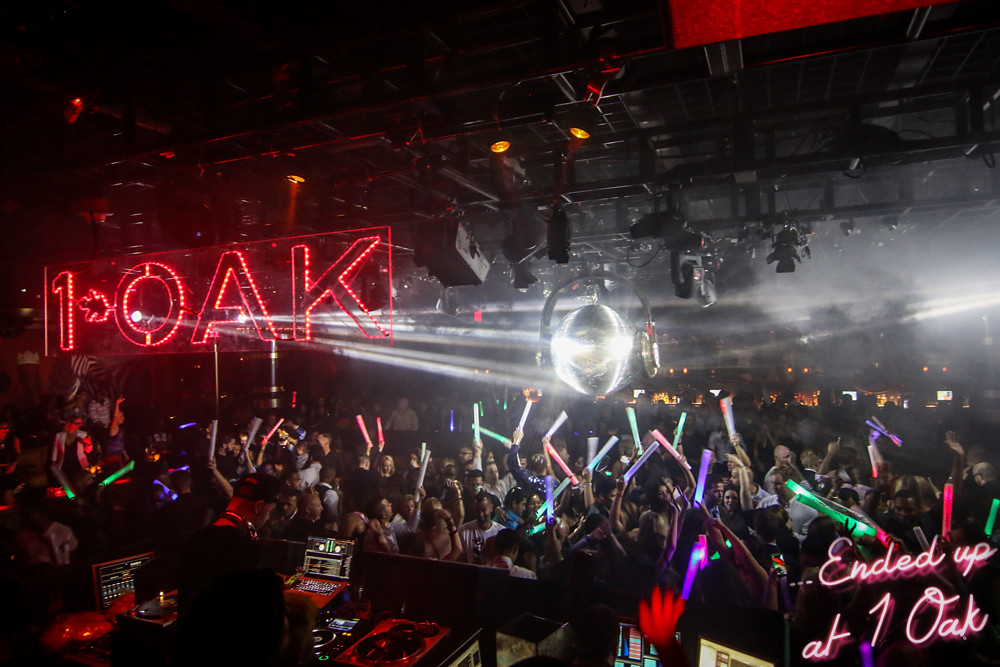This vibrant photograph captures the pulsating energy of an indoor nightclub venue. Taken from the DJ's point of view, the image showcases a bustling scene centered around the DJ, who is dressed in all black, including a black hat, and is stationed next to his DJing equipment, complete with spinning discs. Directly in front of him, a large crowd of enthusiastic club-goers dances beneath a misty haze, waving colorful neon glow sticks in hues of blue, green, red, and purple. High above the crowd, various colored lights illuminate the scene, converging on a shimmering silver disco ball that hangs prominently from the ceiling. The disco ball appears almost magical, refracting beams of light across the room. A clear sign on the left side of the image reads "One Oak," confirming the location. The photograph captures the club's vibrant atmosphere in vivid detail, from the intricate metalwork of the lighting rig overhead to the disco ball adorned with over-the-ear style headphones. In the bottom right corner, neon lettering proclaiming "ended up at One Oak" adds a final touch of authenticity to the lively scene.